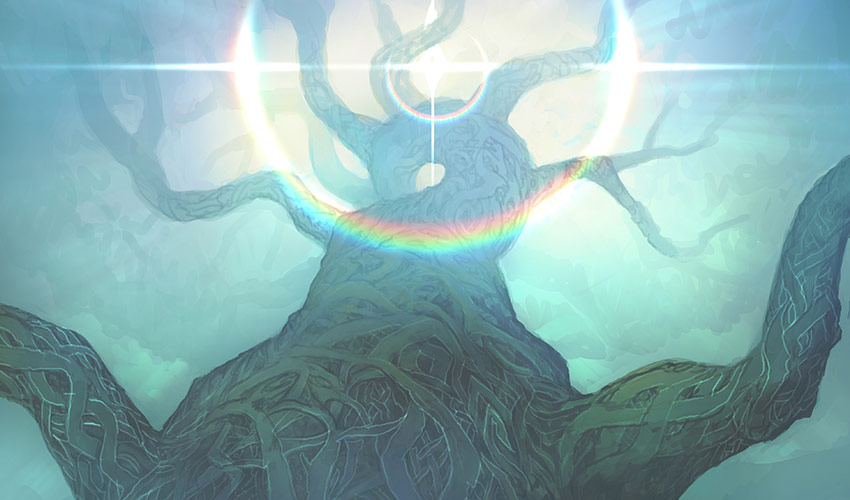This artwork is an abstract illustration of a tree, viewed from beneath as if lying on the ground, gazing skyward. The tree trunk, intertwined with vine-like structures, spirals upward in a helix pattern. Near the base, sturdy branches extend oppositely: two large ones jut outwards to the left and right. Higher up, more branches proliferate, some splitting into smaller, squiggly offshoots. The trunk's swirling design accentuates its upward journey, contributing to a serpentine, almost Medusa-like appearance with branches sprouting intricately in various directions.

The color palette predominantly features shades of green, brown, and teal. The tree itself is rendered in greenish-brown hues, blending subtly into the slightly lighter teal background. This background gradually fades, giving a washed-out effect that reinforces the ethereal quality of the image.

At the top of the composition, the sun glows with a refracted, rainbow-like halo, a circular burst of light painted in reds, greens, and blues. This bright circle is partially eclipsed, its crescent remaining visible, while smaller concentric circles of light extend outward and cross over the top half of the image. Wisps of greenish-brown clouds hover around, adding to the fantastical, surreal ambiance. The scene has a dreamy, science-fiction feel, evoking both natural beauty and otherworldly fantasy.